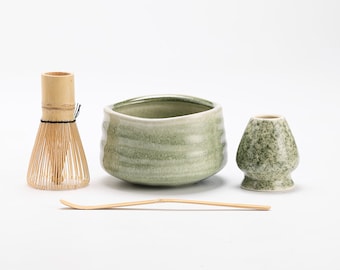This photograph showcases a collection of Japanese-inspired ceramic eating utensils arranged on a white background. On the left, there's a bamboo-colored, triangular bowl, possibly designed to hold sake. Adjacent to it, there is a greenish-gray bowl, with an uneven, handmade appearance and a silver-green interior, perfect for eating from. To its right stands another container, also green but speckled with black, appearing somewhat like a short, rectangular candle holder and likely to be used for drinking sake. In front of these objects lies a thin, bamboo-colored spoon or stirring rod, which gently curves upward, adding to the traditional aesthetic of the set. The overall arrangement exudes an organic, artisanal charm, underlined by the earthy tones and natural textures of the ceramics.